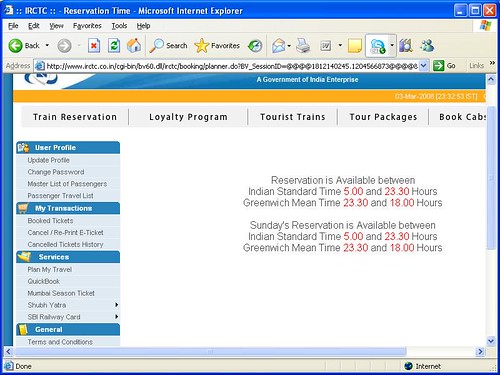This screenshot depicts a web page from a site called RCTC, specifically designed for making train reservations. The displayed title reads "Reservation Time - Microsoft Internet Explorer," indicating the page is viewed on that browser. The site, known as Reservate R, appears to offer various travel-related services. 

The main purpose of the page is train reservation management. Users can access a loyalty program, book tourist train packages, and even arrange for cab services. It clearly states that reservations can be made between 5 AM and 11 PM Indian Standard Time (IST) and provides the equivalent Greenwich Mean Time (GMT).

Additionally, the site allows users to create a personal profile for frequent use, facilitating the booking, cancellation, and reprinting of e-tickets. Users can also view their ticket history and manage it as needed. 

Several links available on the left side of the page enable users to plan their travel in detail. Features like a guest book and various travel-related links suggest that RCTC, likely a train company, offers not only point-to-point train services but also comprehensive tour packages and specialized tourist trains.